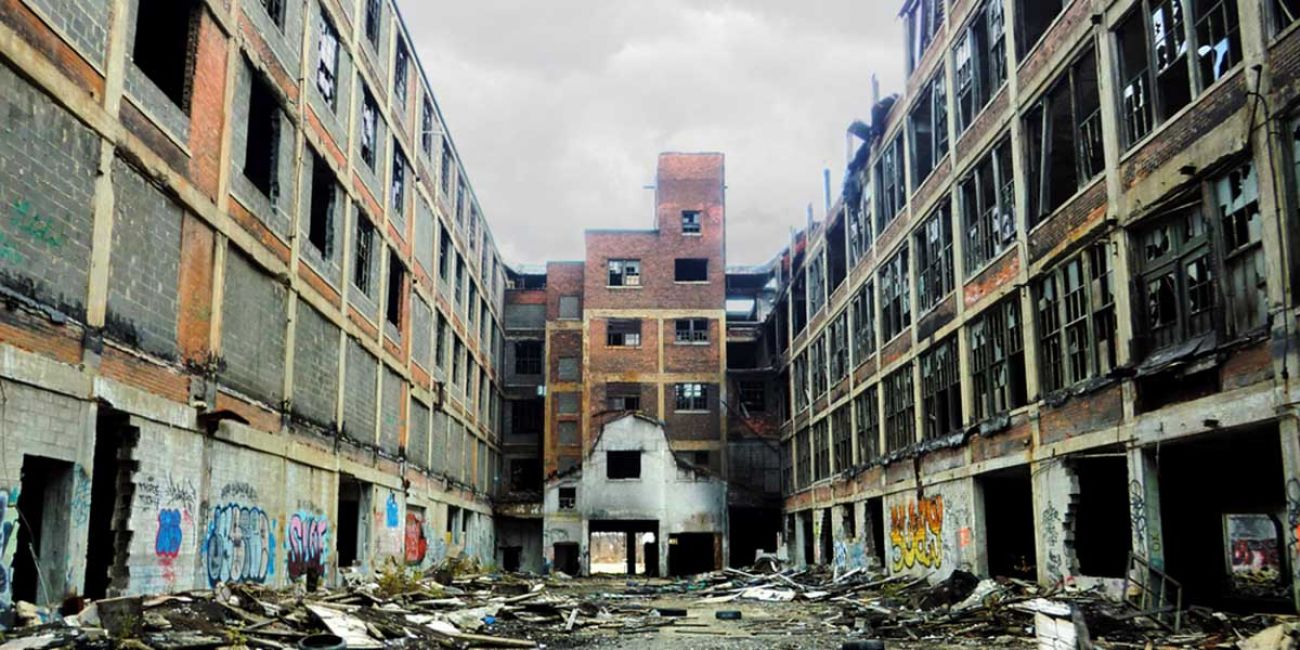The image depicts a scene of urban decay resembling an apocalyptic setting. The focus is on three interconnected buildings, all in a severe state of disrepair. On the left, a five-story red brick building stands, its lower levels marked by gaping holes and gray brick patches covered in indistinguishable graffiti in hues of yellow, blue, pink, and purple. The second, third, fourth, and fifth floors feature a mix of bricked-over windows and smashed glass. On the right, a four-story structure displays more broken, burnt-looking windows framed by red brick. The third building, in the background, connects the left and right structures, completing an alleyway filled with extensive rubble, dirt, and debris. This central building also shows similar decay, including fallen bricks and holes. The remnants of what seems to have been a roof lie scattered on the ground, accompanied by pieces of shattered windows, hinting at a catastrophic event like a fire or explosion. The overall palette is muted, showing mostly rusted brick, weathered wood, and faded graffiti, painting a vivid picture of urban dereliction and destruction.